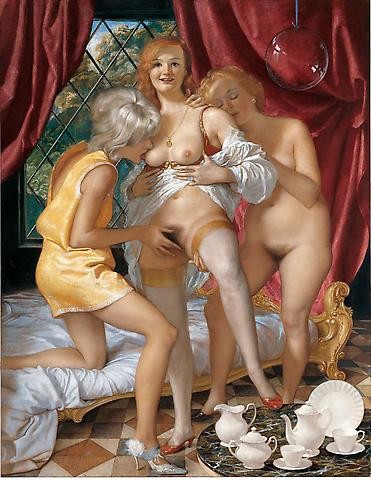This digital artwork, reminiscent of a photo, portrays an intimate and erotic scene with three women in a richly detailed Victorian-era setting. The central figure, a woman with strawberry blonde hair, is shown nearly naked, her red hair cascading over her shoulders. She has slid a red bra below her breasts and discarded white pajamas from her shoulders, exposing her genitals. She is wearing white stockings and red shoes, and smiles directly at the viewer. To her left, a woman with silver hair in a short yellow slip dress and silver high heels is attempting to pleasure her. To the right, there is a fully naked woman with long hair touching the central figure. Behind them, red drapes frame a slatted window revealing an outdoor scene, and a bed with white sheets stands nearby. In the foreground, a detailed black marbleized table topped with a white tea set, including teapots, teacups, and plates, completes the setting.